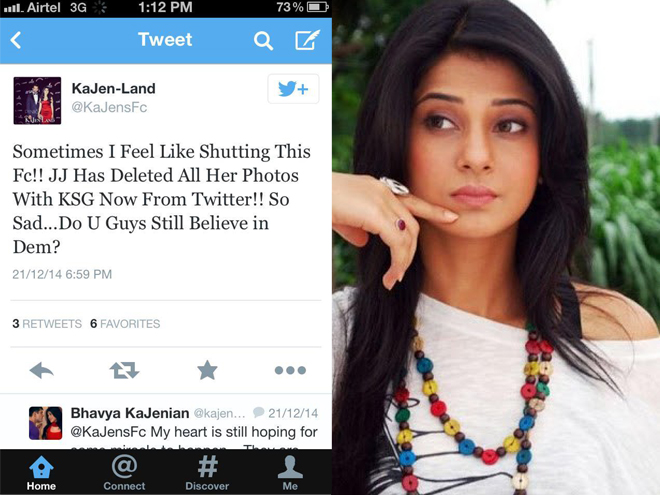The image is divided into two halves. On the left side, there is a screenshot of a tweet from the account "Cajun Land." The tweet, dated December 21, 2014, at 6:59 PM, reads: "Sometimes I feel like shutting this FC. JJ has deleted all her posts with KSG now from Twitter. So sad. Do you guys still believe in them?" The tweet has garnered 3 retweets, 6 favorites, and includes options to select, star, or share. Below the tweet, there is a personal comment from Bavia Kajanen.

On the top left corner, above the tweet, there's an indicator of an aerial 3G phone signal, displaying the time as 1:12 PM and the battery level at 73%.

The right half of the image features a woman with light brown skin and dark brown hair. She is depicted wearing a white shirt and a necklace, looking directly at the viewer.